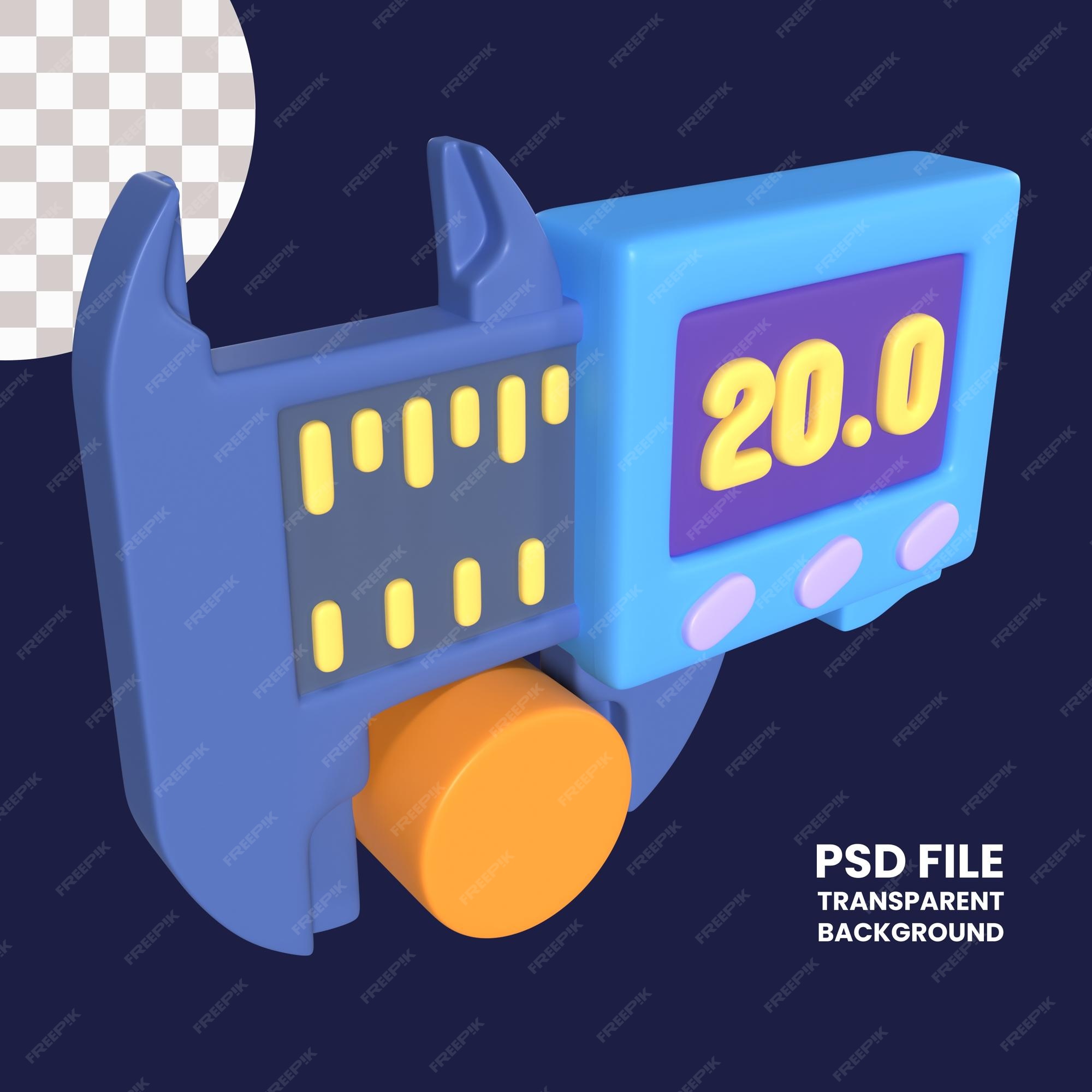This image appears to be a digitally rendered illustration, likely a PSD file designed for educational purposes. The background is dark blue, featuring repeating text that says "free pic," indicative of an openly available example image. The focal point of the image is a peculiar, toy-like object reminiscent of a pair of calipers. The calipers are composed of plastic-like material with sections of light blue and dark blue, almost purple hues. The left segment of the object, which resembles the arms of a wrench, contains yellow, cigar-shaped columns and an orange circular peg at the bottom. The right segment showcases a digital monitor displaying the measurement "20.0," with three pink or purple buttons beneath it. The bottom right corner of the image prominently states "PSD file, transparent background," while a checkerboard pattern of light gray and white squares appears at the top left, further emphasizing the image's digital and editable nature.